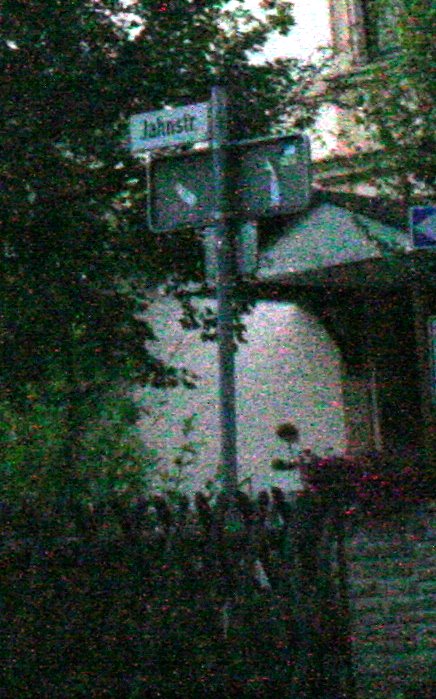This color photograph, presented in portrait orientation, is notably grainy and pixelated, contributing to its overall fuzzy appearance. The image depicts an outdoor scene during daylight hours, as natural light illuminates parts of the setting. In the foreground, there’s a black fence and, behind it, a light gate with plants entwined. A prominent feature of the image is a street sign, partly obscured and facing slightly away. The visible portion of the sign reads “J-A-H-N-S-I-T.” 

Adjacent to this, there's another blue and white sign near a two-story stone building. Outside the building, steps are noticeable, suggesting an entryway, and the area is adorned with green shrubbery, pink flowers, and tall trees, including one with distinctive little red flowers. To the right, a small brick wall and a white awning can be observed in the background, contributing additional architectural details to the scene. The photo, though of poor quality and possibly shot in shaded conditions, captures a quaint residential area, hinting at a serene yet somewhat neglected atmosphere.